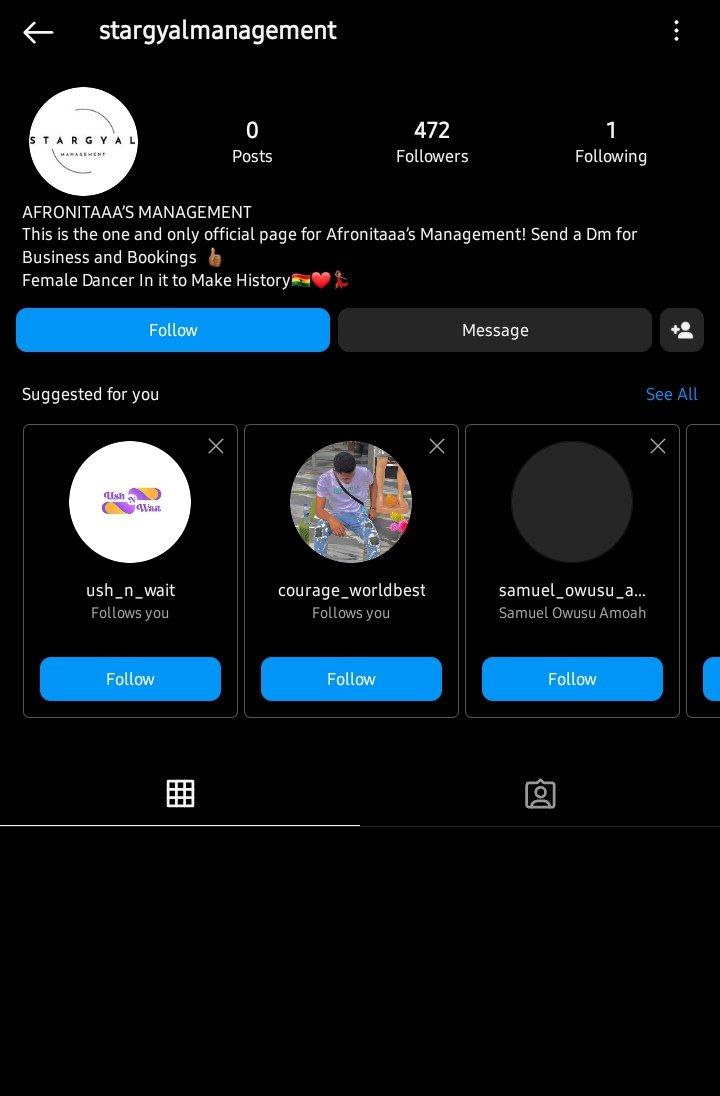The image appears to be a screenshot taken from a mobile phone, featuring a black background. At the top of the screen, in white text, it reads "Star Gail Management." To the left of this text is a left-pointing arrow, presumably for navigating back to the previous screen. On the far right, there are three vertically aligned dots indicating additional options.

Below the header, there is a white circular logo, followed by some key metrics displayed in white text: "0 posts," "472 followers," and "1 following." Additional information, also in white text, is partially visible but not fully readable. 

Beneath these details are three buttons: a blue "Follow" button, a "Message" button, and a button with an icon of a person, the latter two in a lighter shade of black. 

Further down, three square thumbnails are displayed in a row, each with an 'X' in the upper right corner and a circle at the top center. The first square features a white background with a purple and yellow image. The second square appears to contain an image of a person wearing a T-shirt. The third square is a lighter shade of black. Descriptions in white text are written below these squares.

At the bottom of the screen, there is another blue "Follow" button, accompanied by two additional icons.